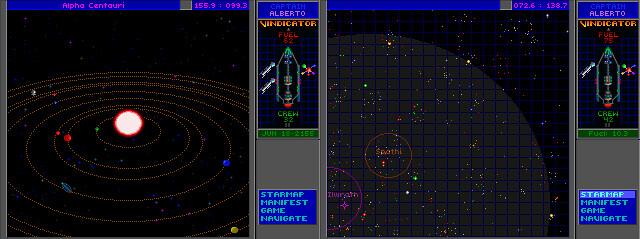This is a vibrant color image possibly part of a video game or computer application interface. The image consists of two adjacent screens with a thin upper border displaying unreadable blue text. Each screen features a grey vertical column on the right side, with the top of each column showcasing a dark blue infographic adorned with various green, red, and white elements, which are indistinct. A blue triangular or rectangular label with white text, including the words "standard" and "game," is also visible.

The left side of the image depicts a solar system model with a central sun surrounded by concentric circles, representing orbits, through which planets are aligned. The background is black, enhancing the visual clarity of the celestial bodies. To the right, a star field is illustrated, also set against a black backdrop. Several stars are encircled in purple, red, and green, indicating points of interest or significance. Overlaying the right-hand star depiction is a faint blue grid, adding a layer of structural detail to the cosmic scene.